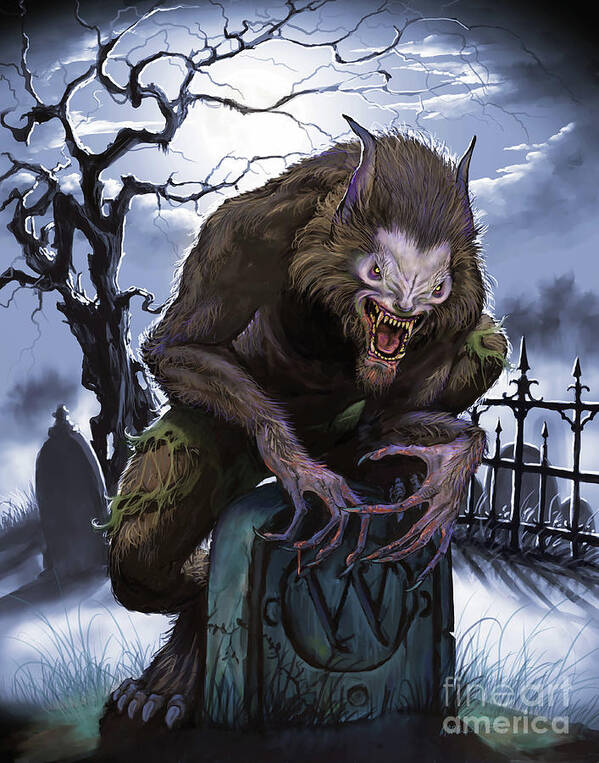The image is a rectangular piece of artwork with the left and right sides being twice as long as the top and bottom. It features a gothic, cartoon-style depiction of a menacing werewolf in a night-time graveyard setting. The werewolf, with brown fur and a white face outlined by its fur, has long, talon-like hands gripping a gravestone, and is posed with one knee on the gravestone and the other leg on the ground. Its open mouth is filled with sharp, yellow fangs, and its eyes are yellowish, enhancing its fearsome appearance. The creature, once wearing green pants that are now heavily frayed, also has long toenails and pointy horns.

The gravestone in the forefront is dark grey, rounded on top, and engraved with a large 'W' inside a circular shape. The background features a moonlit sky shrouded with gray clouds, a gnarly and leafless tree, and a black wrought iron fence, amplifying the gothic atmosphere. In the bottom right corner of the artwork, there is semi-transparent text, potentially a watermark, that reads "fine art America" in lowercase, with "fine art" on one line and "America" just below it.